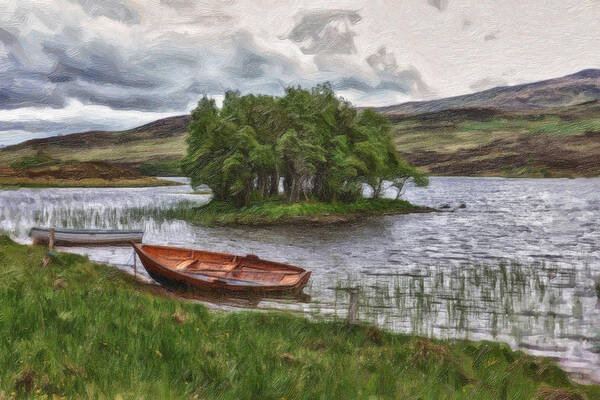This painting depicts a serene outdoor scene centered around a calm lake, which highlights a small island adorned with lush green trees and grass. The lake, with its blue waters, features two rowboats: a brown boat with oars resting near the shore and a blue-and-white boat floating further out. The image is framed by tall green grass and some brown patches in the foreground, indicative of the shoreline from which the scene is viewed. Surrounding the lake is a picturesque mountain range, showcasing a blend of green, brown, and off-yellow hues, adding to the complexity of the landscape. Above, a dramatic overcast sky teems with varying shades of gray clouds, suggesting an impending rainstorm.